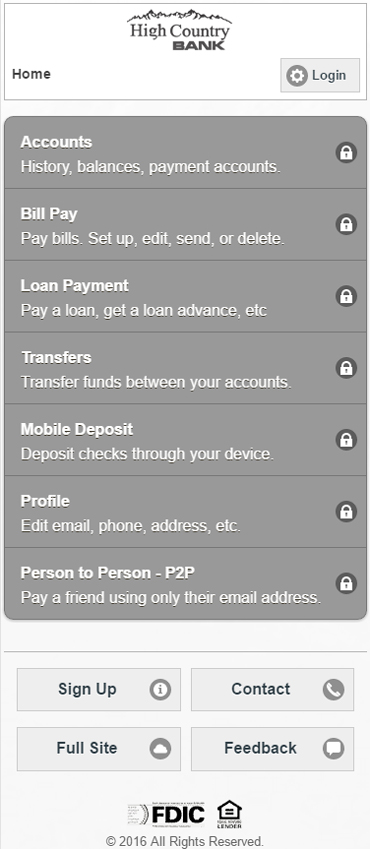This image, taken from a cell phone screen, showcases the interface of the Hi Country Bank's mobile banking application. At the top of the screen, within a white rectangle, "Hi Country Bank" is prominently displayed in the center. To the left, there is a 'Home' button, and to the right, there is a 'Login' button enclosed in a clickable area.

Below this, the interface transitions into a darker gray rectangle featuring a series of options listed in a vertical menu format. These options include:
- Accounts
- Bill Pay
- Loan Payment
- Transfers
- Mobile Deposit
- Profile
- Person to Person (labeled as P2P)

Each option is accompanied by a small lock icon on the right side, indicating secure access. Brief descriptive text appears under each option; for example, under 'Person to Person' (P2P), it explains, "Pay a friend using only their email address."

At the bottom of the screen, there are additional text links for 'Sign Up,' 'Contact,' 'Full Site,' and 'Feedback.' The footer of the screen displays a copyright notice, stating, "© 2016 All rights reserved."